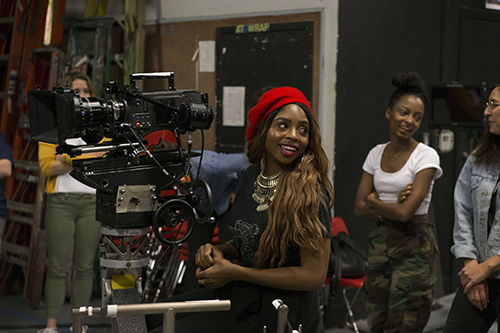The photograph captures a vibrant indoor scene focused on a central female photographer, possibly in a filmmaking class exclusively for women. She is an African-American woman with long hair transitioning from black to brown, wearing a red bandana or beanie, red lipstick, and a black shirt adorned with multiple gold or brown necklaces. She is smiling or speaking while looking to her left, her hands clasped as she operates a large, professional film camera mounted on a dolly. 

The backdrop features a black wall with a bulletin board and a series of colorful ladders, adding a sense of industry and creativity to the scene. To her immediate right, a woman with a white blouse and camouflage pants stands with arms folded, sharing the moment. Another woman in a blue jean jacket, mostly cropped out, can be seen further to the right in a relaxed stance, hands clasped. Further in the background, a woman in a yellow sweater and olive pants is seen near a door and storage area, engrossed in her own tasks. Another woman, dressed in a blue or yellow jacket, white shirt, and green pants, is barely visible behind the camera. This collective moment captures the essence of collaborative learning and enthusiasm in a woman-centric filmmaking environment.